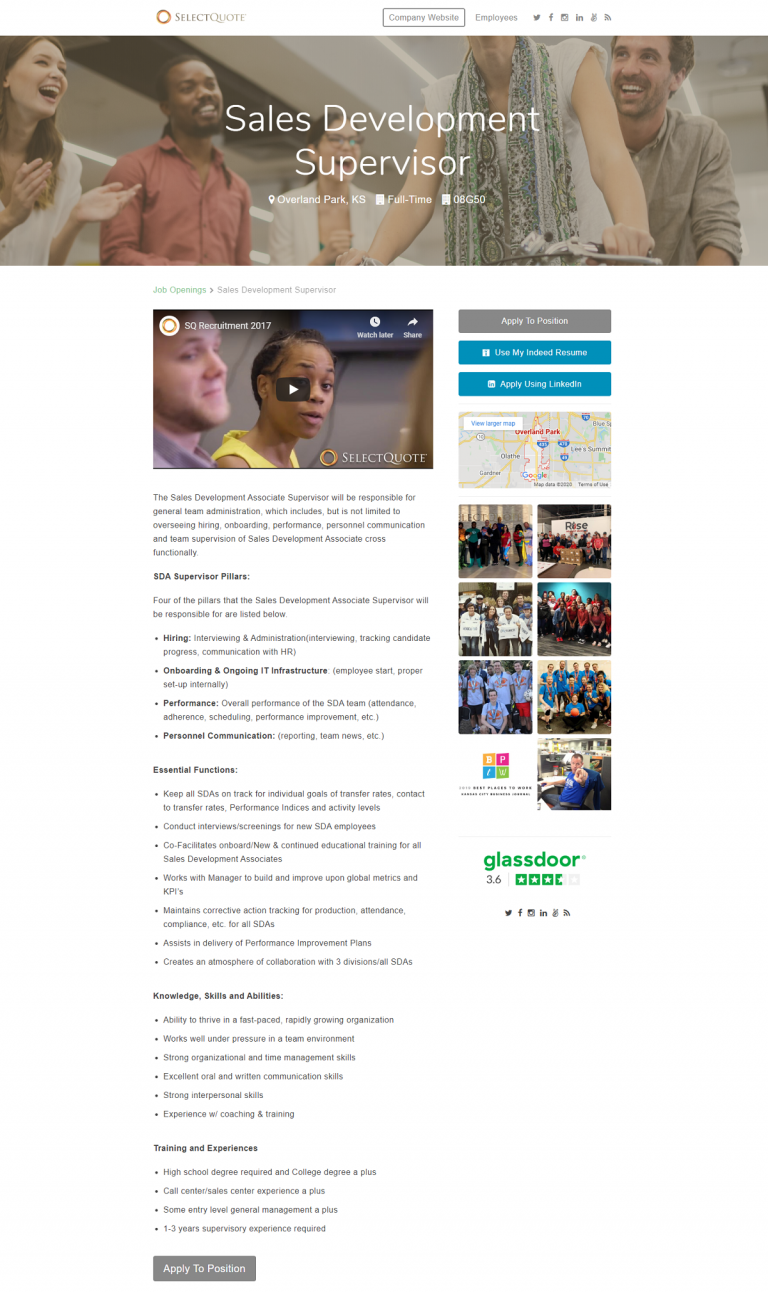Screenshot of a computer or mobile interface displaying a career page with various elements:

- **Top Bar:** A white top bar featuring the Select Quote logo, a gray box with unreadable black text, possibly the word "Extensions," and social media icons.
- **Image Banner:** Below the top bar, there is an image banner spanning across the screen. It depicts four or five people (three women and two men), all smiling, with one person clapping. White text overlaid on the image reads, "Sales Development Supervisor," followed by smaller, unreadable text.
- **Main Content Section:**
  - **Left Side:** A video thumbnail with a play button in the center, featuring a lighter-skinned man and a darker-skinned woman. Below the video, there are several paragraphs of unreadable text, and at the very bottom, a gray "Apply to Position" button.
  - **Right Side:** Next to the video, there's another gray "Apply to Position" button, followed by two stacked horizontal blue buttons with unreadable text. Below these buttons is a small map.
  - Continuing down, there are four rows of images with two images per row (totaling eight images). These images depict various individuals and groups, with the bottom left image being an icon.
  - At the bottom right, there is an advertisement for Glassdoor featuring a 3.6-star rating with green stars, though one star is partially covered. Below this, there are additional social media icons.

This detailed caption encapsulates the structure and content of the screenshot, providing a clear visual narrative.